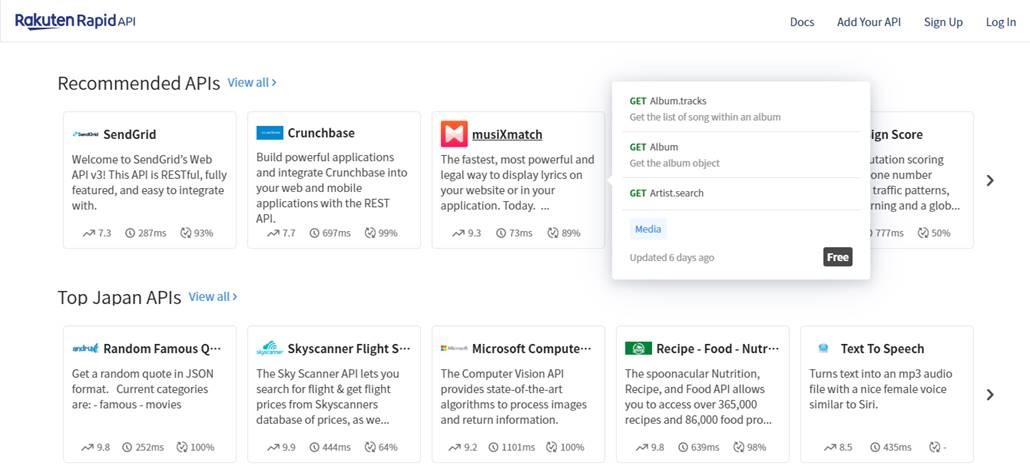**Rakuten RapidAPI Web Interface Screenshot**

The screenshot captures the user interface of the Rakuten RapidAPI website. At the very top, the header displays various navigational links, including options to view "Docs," "Azure API," "Sign Up," "Log In," "Recommended APIs," and "View All."

Below the header, an introductory section welcomes users to SendGrid's Web API version 3. The description highlights the API's RESTful nature, its full features, and ease of integration. Additionally, there are panels showcasing different APIs such as:

1. **SendGrid's Web API v3:** A RESTful and feature-rich API designed for easy integration.
2. **Crunchbase API:** This API empowers developers to create robust applications by integrating Crunchbase data into their web or mobile apps.
3. **Musixmatch API:** Known as the fastest, most powerful, and legal way to display lyrics on websites or applications.

A highlighted window within the interface points specifically to Musixmatch, providing detailed functionalities like "Get album tracks," "Get the list of songs within an album," "Get album object," "Get artist search," with a note stating it was updated 6 days ago and is free.

Further down, several featured APIs are displayed:

- **TopJapan APIs (Random Famous Quotes):** Provides a random quote in JSON format from various famous movies.
- **Skyscanner Flight API:** Allows users to search for flights and retrieve flight prices from Skyscanner's extensive price database.
- **Microsoft Computer Vision API:** Uses advanced algorithms to process images and return detailed information about the visual content.
- **Recipe Food Nutrition API by Spoonacular:** Offers access to over 365,000 recipes and 86,000 food products.
- **Text to Speech API:** Converts text into an mp3 audio file with a female voice similar to Siri.

This comprehensive and well-structured interface indicates a powerful and diverse platform designed to cater to various API needs, ensuring seamless integration and functionality for developers.